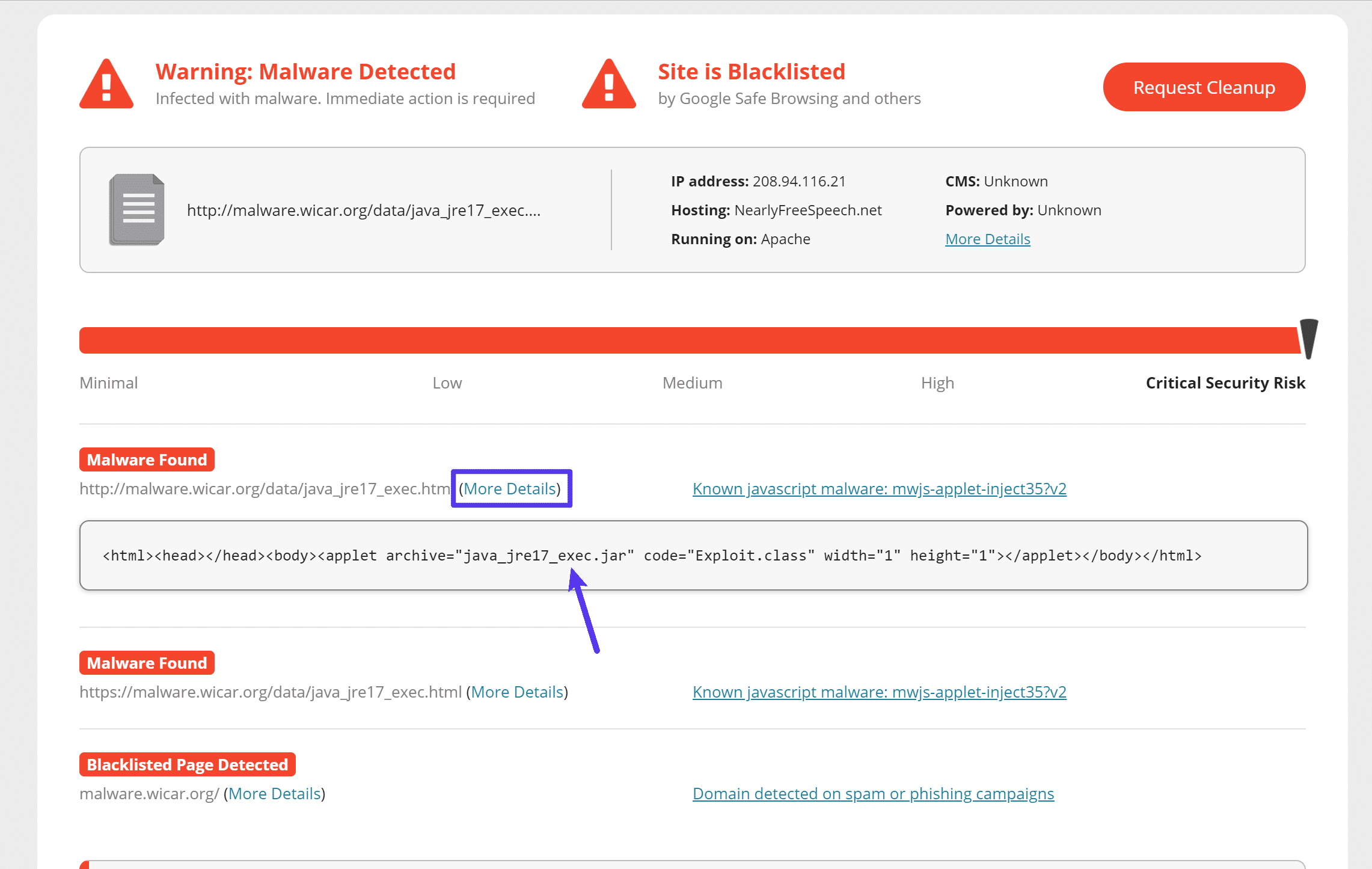The image displays a warning web page indicating a malware alert. The page is framed by a light gray border and features a stark white background with prominent red headers. Across the top in bold, red letters, it declares "WARNING: Malware Detected," accompanied by a red triangle with a white exclamation mark. Below this, another statement reads, "Infected with Malware – Immediate Action Required," with a similar red warning triangle. Adjacent to this, another alert in red states, "Site is Blacklisted by Google Safe Browsing and Others," next to yet another warning triangle.

To the right, there is a prominent red button labeled "Request Cleanup." Beneath these warnings, a pale gray text box displays a URL: "malware.wicker.org/...," followed by details including the hosting IP address and partial hosting information, suggesting the server is associated with "nearlyfreespeech.net" and utilizes Apache. The content management system (CMS) is listed as unknown, and there's a blue, underlined hyperlink for "More Details."

Further down, a horizontal red bar with a black, downward-pointing triangle acts as a security risk indicator. The spectrum ranges from "Minimal" to "Critical," with the indicator pointing towards "Critical." Intermediate levels are marked as "Low," "Medium," and "High."

On the left, another red button is labeled "Malware Found," followed by a URL. A cobalt blue rectangle surrounds a "More Details" link for additional information. This section also mentions a specific type of malware: "Known JavaScript Malware Applet Injected." An underlined "More Details" link suggests further information is available. Additionally, there is a notification of another type of JavaScript malware and that the page has been blacklisted. The bottom of the page appears truncated, indicating that more content or detailed information is available via scrolling.